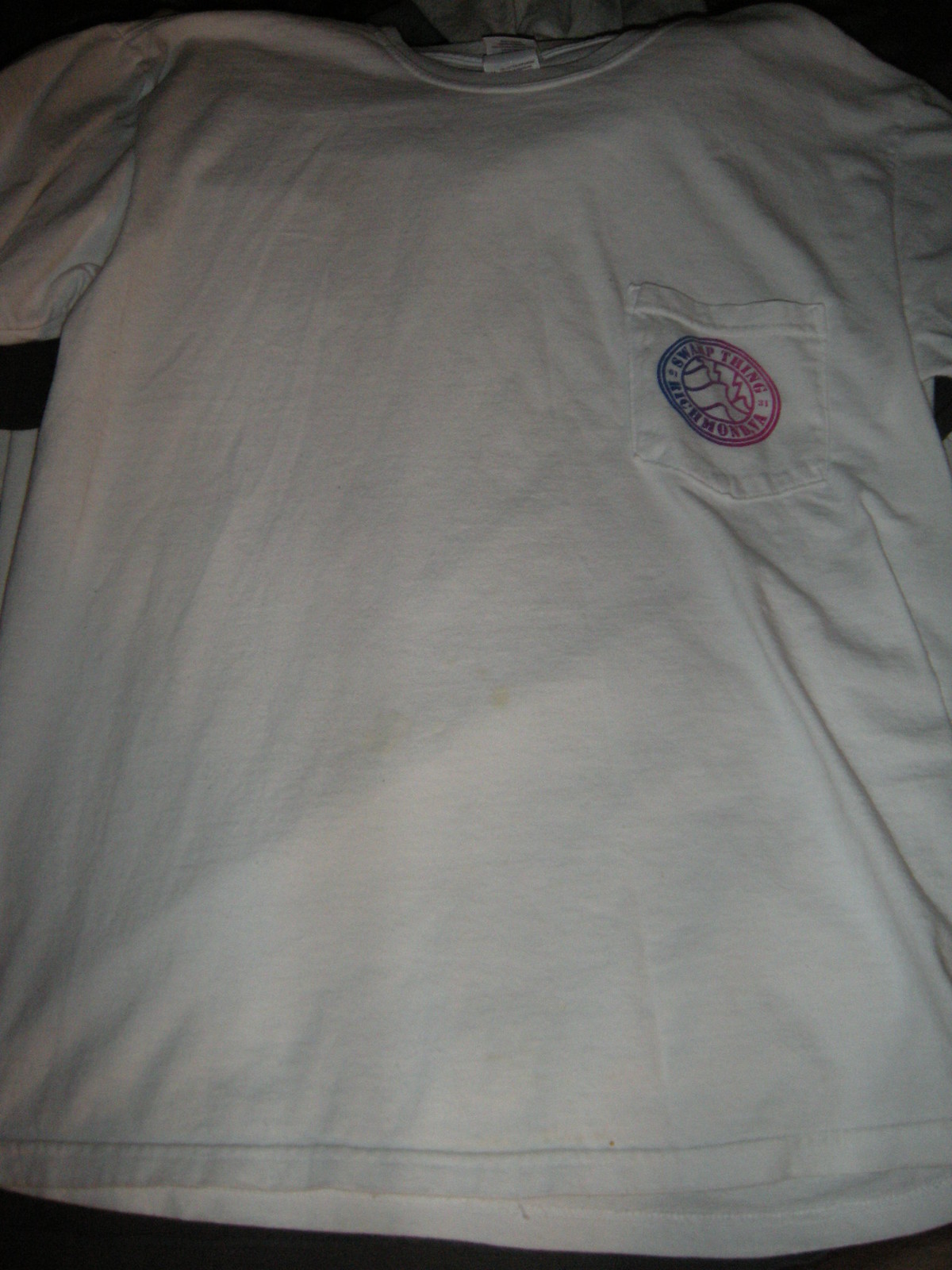This image captures a worn, white cotton t-shirt laid flat on an indeterminate dark surface, likely illuminated solely by the camera's flash, resulting in minimal lighting. The t-shirt is wrinkled and creased, indicating it hasn't been ironed. The collar of the shirt, a standard round-neck design, appears at the top of the image, aligned diagonally with the tag flipped up inside. Each sleeve extends out of the frame, suggesting the shirt's substantial spread. The t-shirt features a pocket located midway on the right side, with a circular, multicolored logo comprising blue and pink hues. The logo includes the text "Swamp Thing" in a semi-circular pattern at the top and "Richmond, VA" at the bottom, with an interior design resembling mountains or lines. Additional details include faint dirt or food marks scattered across the fabric, hinting at the shirt's used condition.